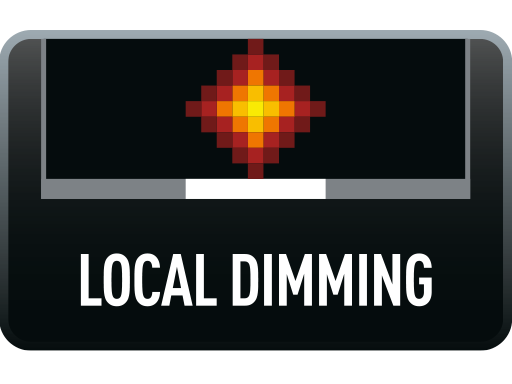The image is a detailed graphical drawing of a rounded rectangle with a gradient background transitioning from black at the bottom to a lighter gray at the top. Inside this primary rectangle, there is a secondary rectangle with a light gray border and a black internal background, centrally featuring a pixelated diamond shape. The diamond shape starts with a yellow center and radiates outward in progressively darker squares of orange, red, and a deep maroon, resembling a mosaic or pixelated sun. A thin gray line runs from the top, dividing the inner rectangle, and across the bottom, white capitalized block letters display the text "LOCAL DIMMING."